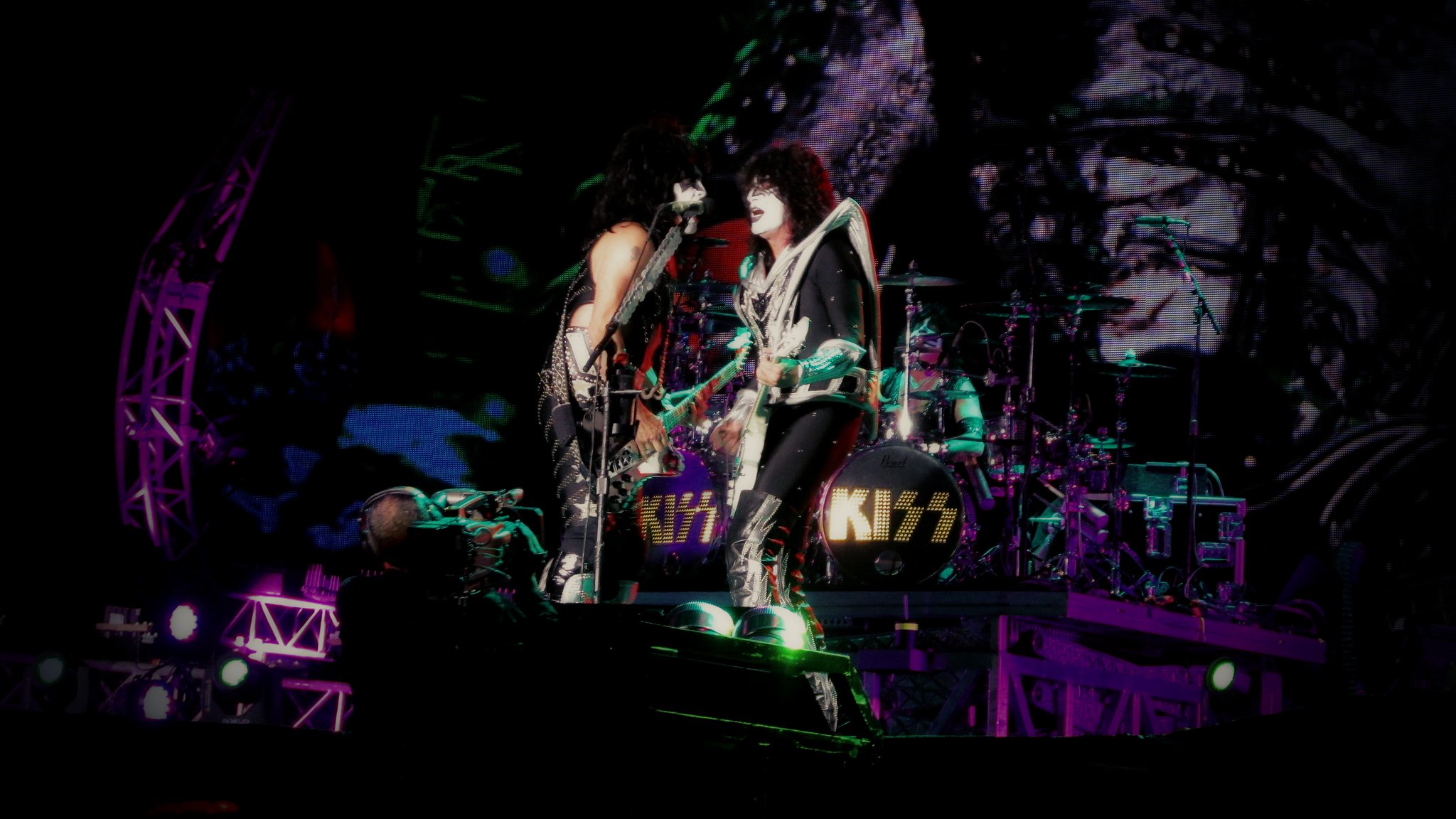This grainy, fisheye-lens image captures the iconic band KISS performing live on stage, seemingly from a first-row crowd perspective. The stage is warped to the left, with scaffolding intricately lit in purple. Paul Stanley stands out in sharp focus, capturing the attention as he passionately sings into a microphone while holding his guitar. Dressed in a black bodysuit with striking thigh-high black boots and large silver shoulder pads, his look is completed by his signature white face paint and long curly hair. To his left, Gene Simmons, clad in a sleeveless black bodysuit, faces away but is engaged with his guitar, his white face paint with a black star around his eye also prominent.

In the background, the drummer energetically plays a drum set emblazoned with "KISS" in large gold letters. The stage lighting casts a vivid purple hue across most of the scene, contrasting with a bright white spotlight illuminating Paul Stanley and Gene Simmons. Additionally, a shadowy figure believed to be a cameraman can be seen pointing a camera towards the performers. A faint video montage plays in the pixelated dark background, contributing to the enthralling and eclectic ambiance of the concert.